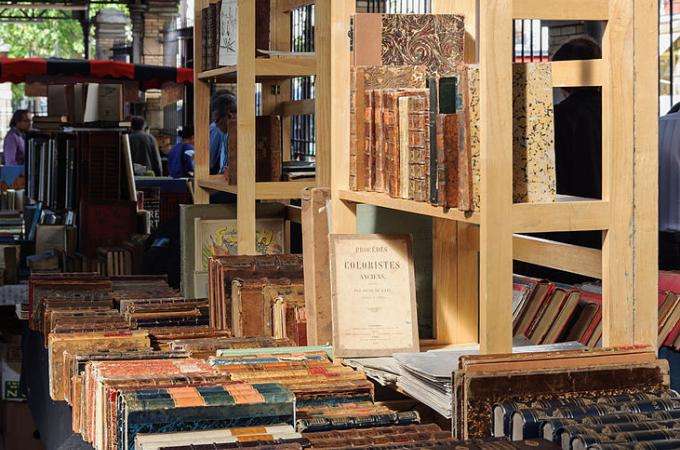The image captures an interior room filled with numerous wooden bookshelves, giving it the appearance of a traditional library. The shelves, all elegantly crafted from wood, are meticulously lined with an assortment of books and files, lending an air of old-world charm to the space. In the distant background, vague silhouettes of people can be seen, though their identities are indiscernible, obscured by the myriad of shelves that dominate the room. The horizontal photograph artfully showcases the intricate layout and timeless ambiance of this literary sanctuary.